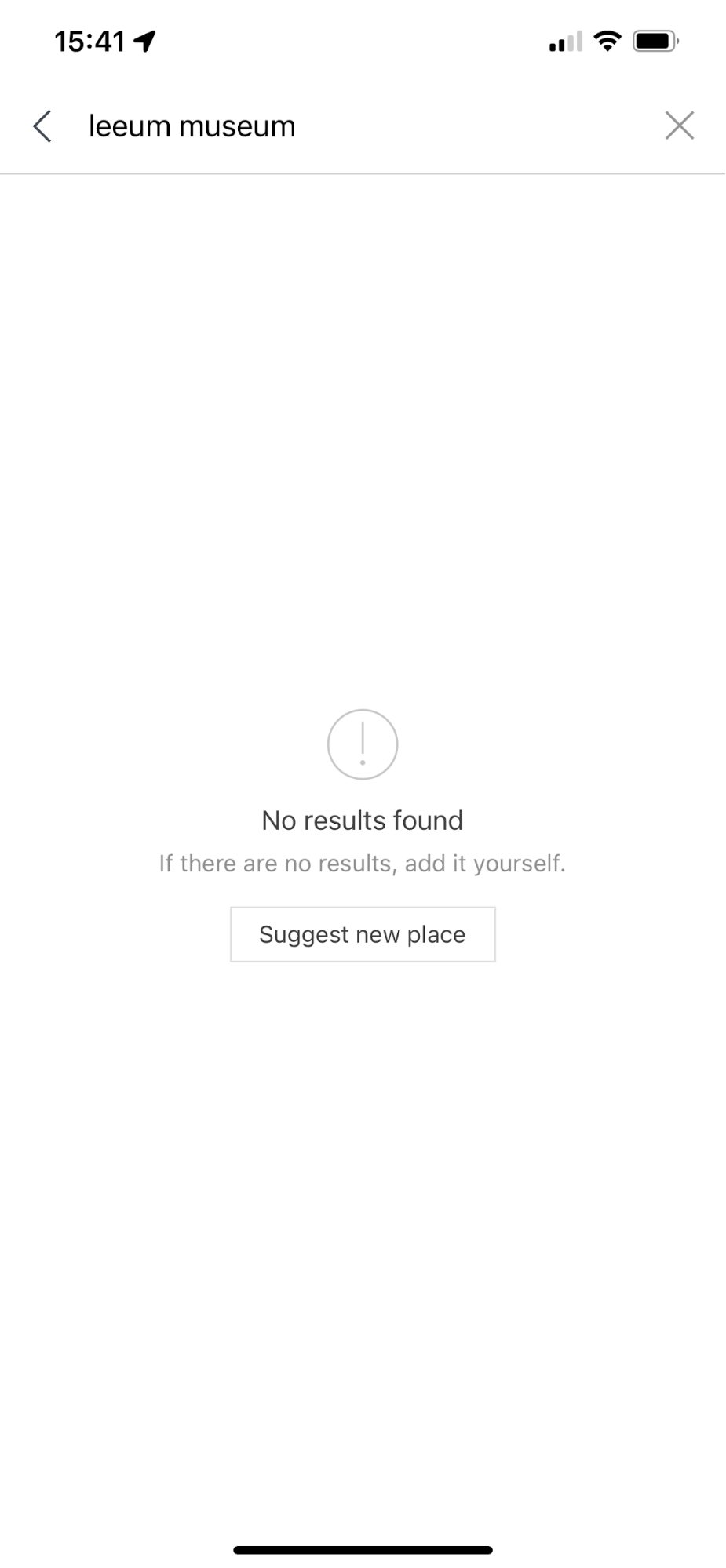This screenshot, taken from a smartphone, displays a web search interface with a clean, white background. In the upper left corner, bold black text indicates the time as 15:41, accompanied by a directional arrow pointing toward the upper right. Adjacent to this, three icons are displayed: a bars indicator showing connectivity strength, a Wi-Fi icon, and a battery life indicator. 

Centered below the status bar is the search bar, flanked on the left by a directional arrow pointing left and containing the search term "Liam Museum." On the far right of the search bar is a small 'X' icon for clearing the search. Directly beneath the search bar is a thin, light gray line extending horizontally across the screen.

The main content area is largely blank, dominated by a central feature: a light gray outlined circle containing an exclamation mark. Below this symbol, black text declares "No results found." Further down, in darker gray text, a suggestion prompts, "If there's no result, add it yourself." At the very bottom of the display, there is a light gray-outlined rectangle containing black text that reads, "Suggest new place."